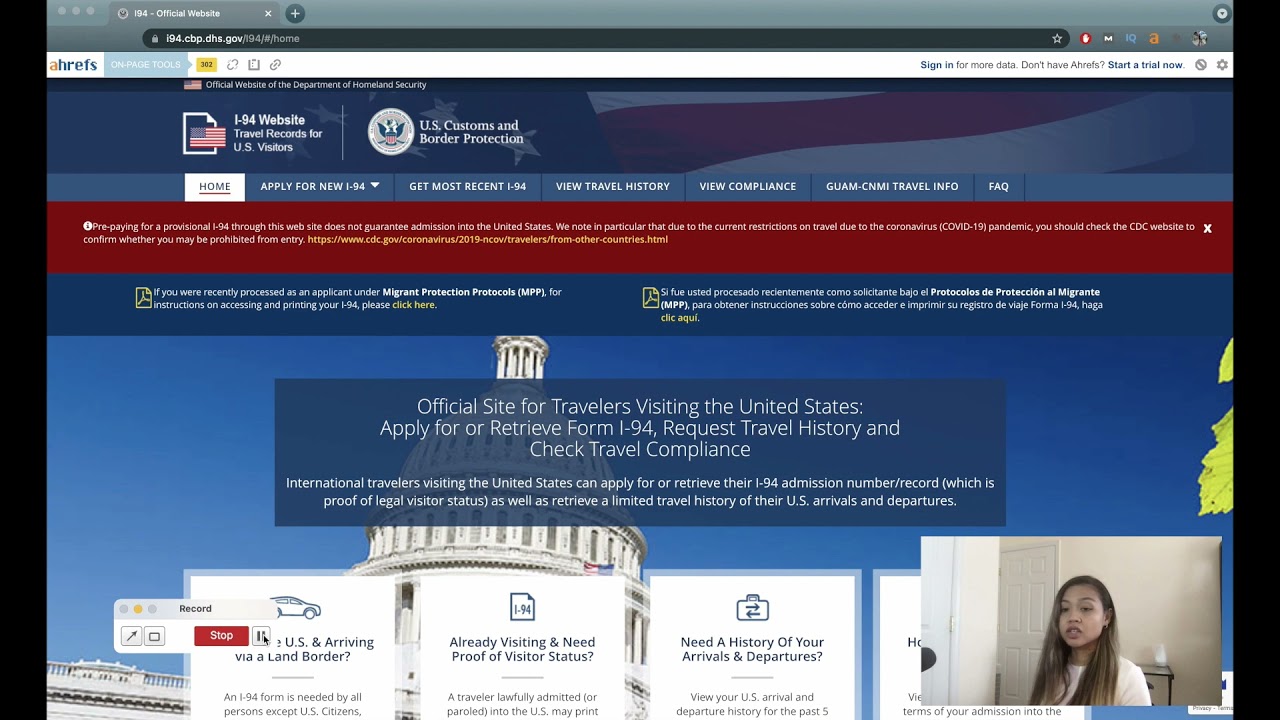This image depicts a detailed view of the I-94 website, which is dedicated to travel records for U.S. visitors. Prominently featured is an advisory that emphasizes the importance of checking the CDC website for up-to-date information on travel restrictions related to the ongoing coronavirus pandemic. The webpage serves as a crucial resource for travelers, offering essential information regarding entry and exit records. The repetitive focus of the image on ensuring visitors check the latest travel guidelines highlights the evolving nature of international travel in response to health concerns.